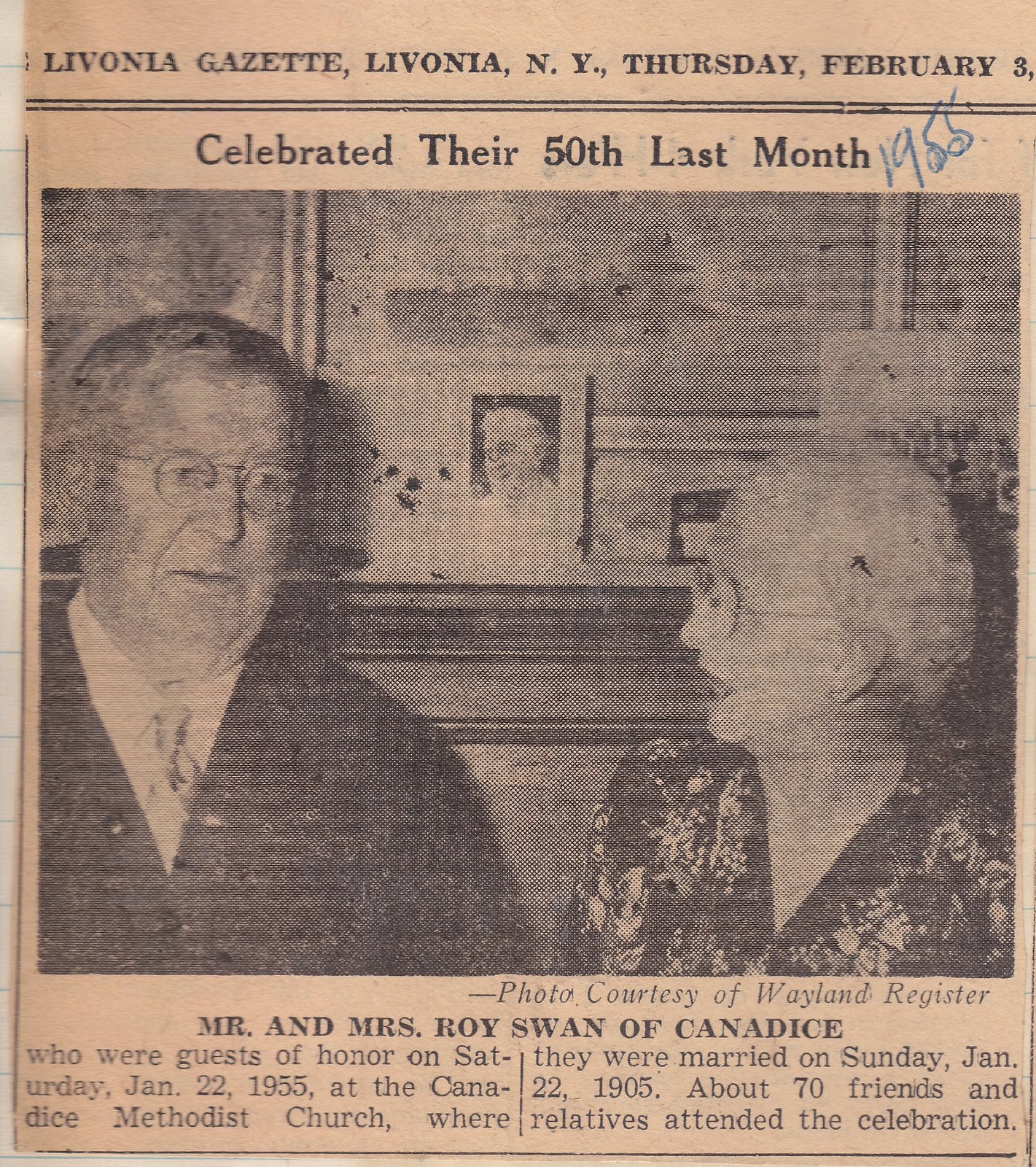The image is a black-and-white newspaper clipping from the Livonia Gazette, Livonia, New York, dated Thursday, February 3rd, 1955. The headline reads "Celebrated Their 50th Last Month." It features a vintage black-and-white photograph of an elderly couple, Mr. and Mrs. Roy Swan of Canadice. The husband stands on the left, gazing off to his left, while his wife stands to his right, looking at him. She is adorned in a print dress and glasses, with white hair. In the background, they stand in front of a paneled wall with some photographs visible on a countertop. The caption below the photo states that they were guests of honor on Saturday, January 22, 1955, at the Canadice Methodist Church, where they had been married on Sunday, January 22, 1905. Approximately 70 friends and relatives attended the celebration. Additional text below the photograph notes that the photo is courtesy of the Wayland Register. The clipping is characterized by its tan, black, blue, and various shades of gray and white, reaffirming its vintage newspaper style.